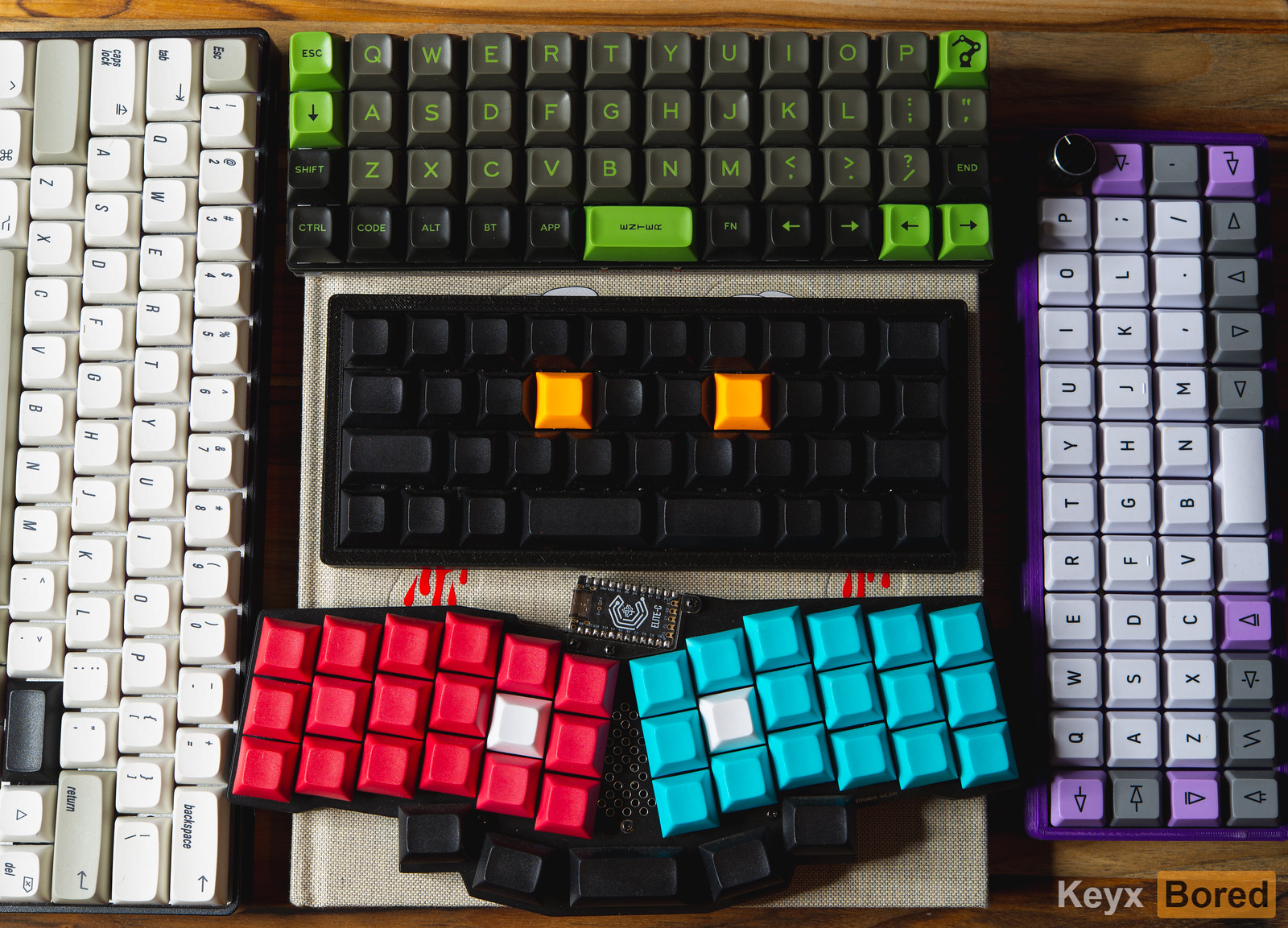This bird's-eye view photograph captures a collection of various mechanical keyboards arranged on a wooden desk. In the lower right corner, the text "K-E-Y-X" in white and "B-O-R-E-D" in black is displayed within a small orange rectangle. Starting from the left, there is a white keyboard featuring black letters and numbers on the keys, with one black key and a couple of gray keys turned sideways. In the upper center of the image, a black keyboard with vivid neon green letters, numbers, and function keys, including a neon green space bar and arrows, stands out prominently. Directly below it, another black keyboard is visible, distinguished by two larger orange keys in the middle. Scattered below that are individual blue and red keys, with occasional white keys interspersed. Towards the bottom middle of the desk, a uniquely shaped squiggly keyboard with alternating blue and red keys appears. Finally, on the right side, a keyboard sporting a mix of light purple, white, and gray keys with black text can be seen, with the backplate of the keyboard being purple and the layout turned sideways.